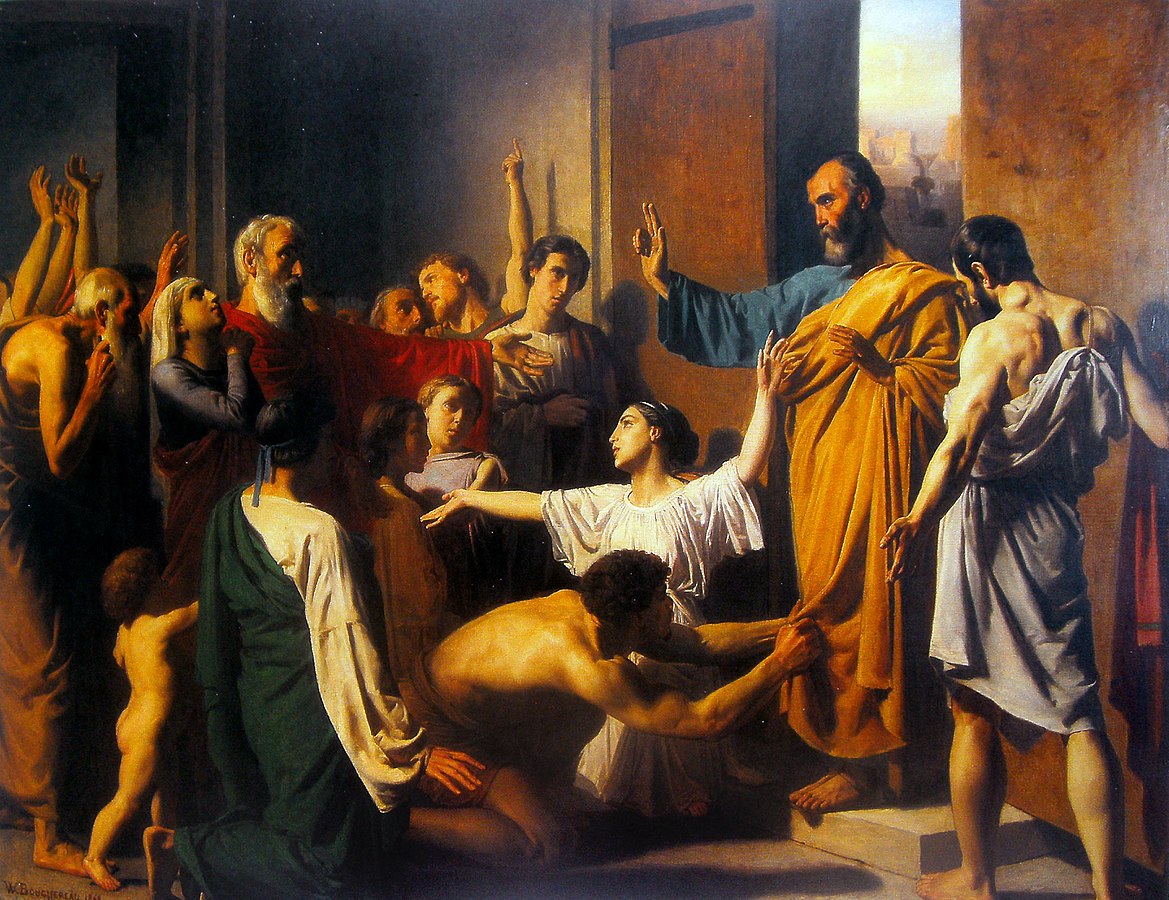This detailed and realistic painting depicts a scene from ancient times, reminiscent of the Renaissance or perhaps classical Greek art, characterized by the elaborate and historical attire of the figures. Central to the composition is a tall, bearded man, draped in a blue tunic beneath a golden robe, who stands authoritatively with his right hand extended, two fingers raised in a gesture that suggests he is addressing the crowd before him. This dominant figure appears to be a prophet or a significant religious leader, as suggested by the reverent attention of the surrounding people.

The crowd comprises individuals dressed in simple robes and tunics, many of whom are either kneeling or standing with their hands raised towards the central figure, highlighting their veneration. Among them, at the feet of the bearded man, is a nearly naked man clutching at the hem of the golden robe, and a young woman in a white dress, also kneeling in supplication. A small naked child is present at the bottom left of the scene, contributing to the theme of humility and vulnerability among the followers.

In the background, partially open brown doors reveal a glimpse of the outside world, with a distant city visible under daylight, adding depth and context to the indoor setting. The room itself is dimly lit with an orange glow, emphasizing the use of light and shadow to create a realistic and dramatic atmosphere. The intricate details and the expressions of the figures make this painting a profound representation of a historical and possibly religious moment, capturing the intense emotion and the solemnity of the scene.